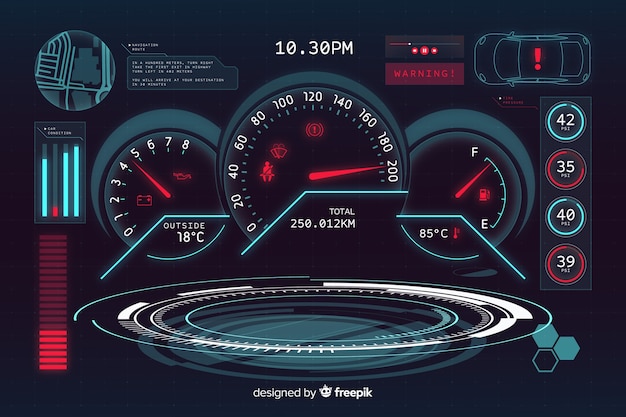The image is a detailed digital graphic resembling a car’s diagnostic screen with a black background. At the center, there are three main gauges: the middle gauge, likely a speedometer, ranges from 0 to 200 with a red needle pointing near 200. Below it reads "Total 250.012 km." The left gauge appears to be a battery meter ranging from 0 to 8, with a red needle between 4 and 5, and icons for the battery and oil indicators. Below this, it says "Outside 18 degrees Celsius." The right gauge looks like a fuel gauge, marked from F (full) to E (empty), with a red needle near F and a red gas pump icon. Below reads "85 degrees C." 

Additional elements include a top bar with "10:30 p.m." centered, and an image of a car at the top right with an exclamation point warning light. Below this are vertical meters in blue and red colors, marked with numbers including 42, 35, 40, and 39. The screen displays various readings in subdued bluish-green, bright red, and white colors. A circular mini-map appears at the top left. At the bottom, it states "Designed by Freepik."